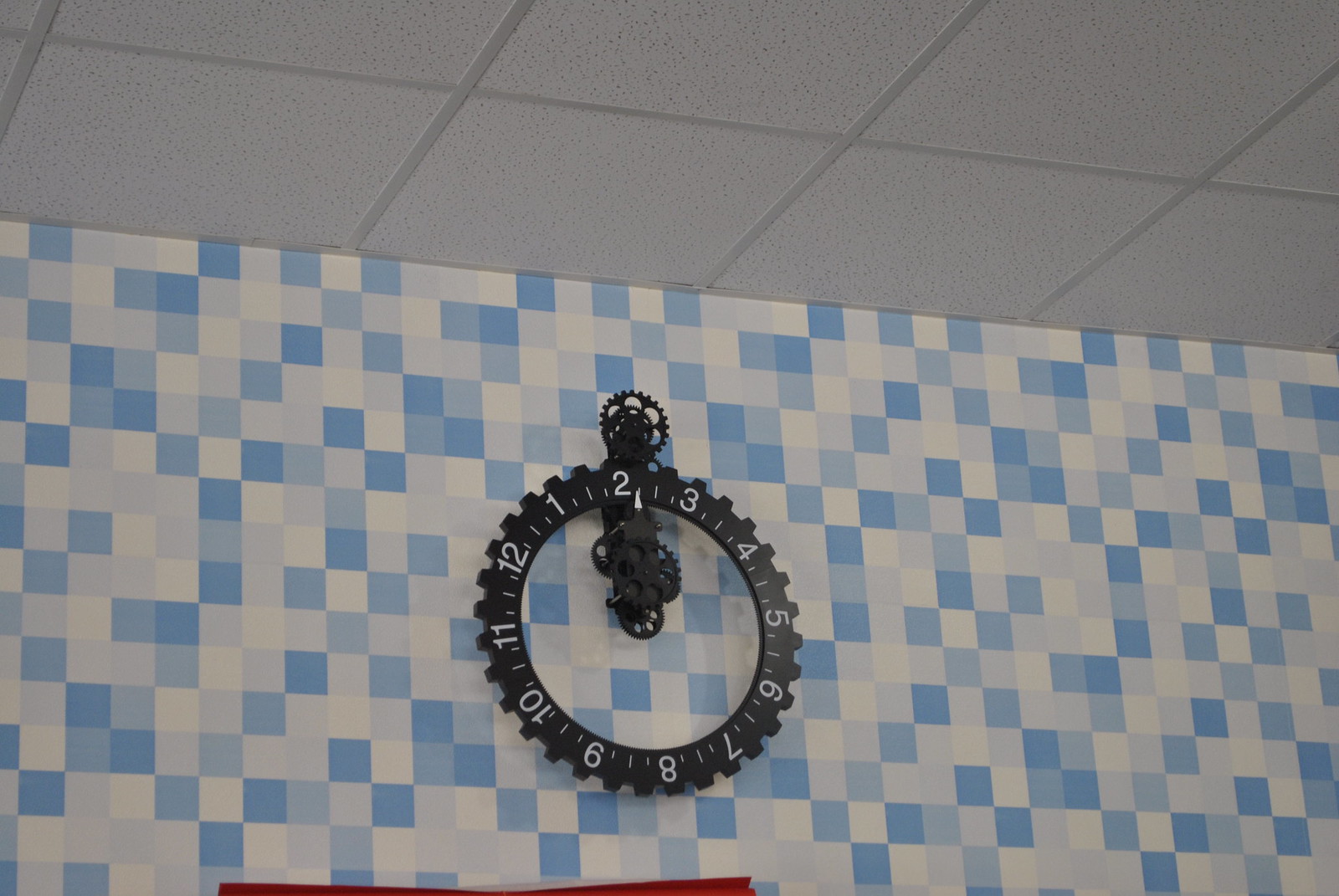The image captures a segment of a room showcasing both the ceiling and part of a wall. The ceiling is a standard drop ceiling with white, foam-textured tiles neatly placed within a lighter-colored grid, commonly used in offices and commercial spaces for easy access to wiring and ventilation. 

The adjacent wall features an eye-catching, multi-colored checkerboard pattern of wallpaper, incorporating shades of white, light blue, dark blue, gray, and light gray in a harmonious arrangement. This intricate design serves as an interesting backdrop for a uniquely styled wall clock positioned centrally within the frame. 

The clock is designed to resemble a series of interlocking gears, with a smaller gear-like structure at the top and a larger gear forming the clock face. The mechanism looks as though the gears turn to indicate the time. At the moment captured, the number '2' is prominently displayed at the top of the clock face, with additional gears visible in the center. A small white arrow is positioned, pointing directly at the '2', suggesting it is 2 o'clock. The overall composition showcases a blend of utilitarian ceiling design and creatively patterned wall decor, anchored by the visually intriguing gear-themed clock.